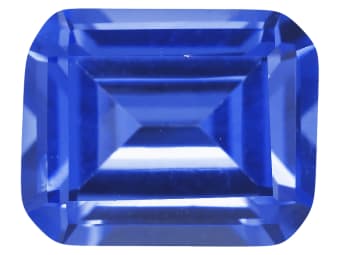This high-resolution image features a meticulously crafted blue gemstone set against a pristine white background. The gemstone, likely photorealistic but possibly digitally rendered, is rectangular with softened, rounded corners. Its surface is intricately detailed with beveled edges and etched squares, creating an impression of depth and dimension.

The geometry of the gem includes a rectangular border encasing a recessed inner rectangle, adding to its layered appearance. The shades of blue transition from nearly black at the edges to very light hues in the center, enhancing the stone's three-dimensional look. A reflective white streak can be seen in the lower right portion, indicating a light source's reflection.

The upper right corner of the gemstone exhibits a gradient from black to dark blue, then gradually lightening down the right edge. The interior showcases a complex pattern of dark and light blues interspersed with whites, reminiscent of a deep, multi-faceted sapphire. Wet spots of white suggest a glossy, polished finish, adding to the gemstone's allure.